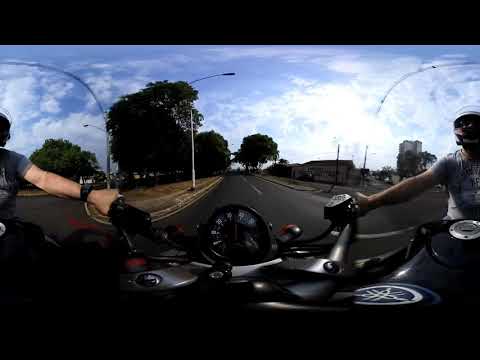In this 360-degree photo, we see a person, wearing a helmet and likely sunglasses, gripping the handlebars of a mostly black motorcycle. The individual is wearing a gray t-shirt and a watch on their left wrist, indicating it's a warm, sunny day. The image, taken from the perspective of the rider, features the motorcycle's dashboard at the bottom center. The background includes trees, buildings, a street with a median, and a partly cloudy sky with sunlight in the top right corner. The photo also frames the scene with a solid black border at the top and bottom, encapsulating the outdoor setting on a paved street lined with a street light amidst a palette of colors including black, blue, white, gray, green, red, and tan.